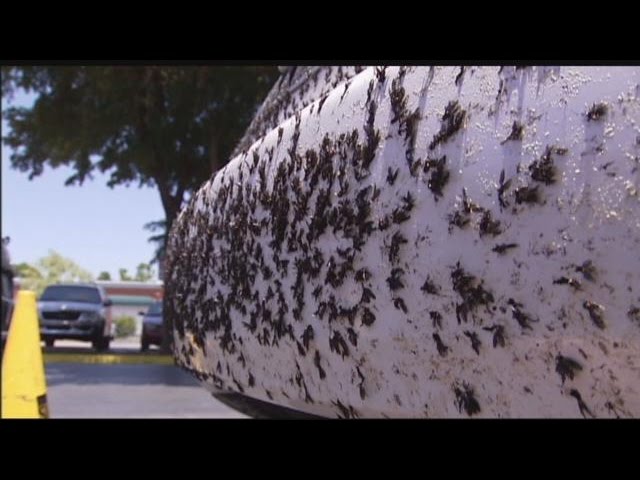The photograph showcases a close-up view of a white car's bumper, heavily covered with a dense layer of various dead bugs, primarily brown and black in color. The aftermath of what appears to be a lengthy and fast journey through a swarm of insects is vividly evident, with areas so densely packed that the white paint of the bumper is scarcely visible. Additionally, some sand is stuck to the bumper, enhancing the impression of a tough trip. A yellow traffic cone is situated to the left of the bumper, indicating a parking lot environment. In the background, blurred but distinguishable, are cars parked under a tree and a building featuring multicolored stripes, possibly a gas station, further setting the scene. The sheer number of insects—estimated to be in the hundreds—splattered across the bumper is particularly striking.